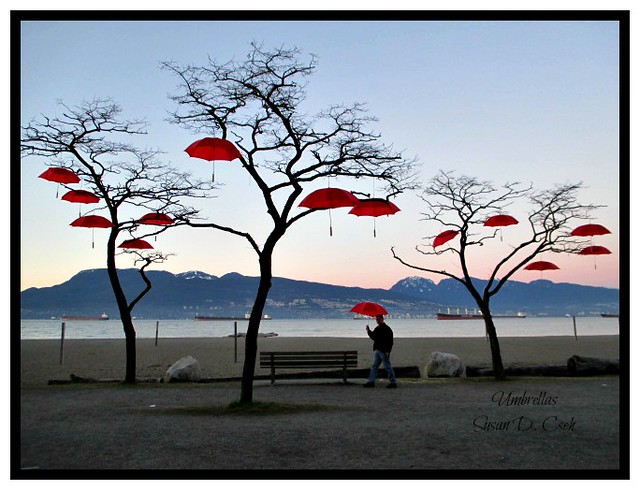In this enchanting photograph, taken by Susan D. Cook and subtly marked with "Umbrellas" in the lower right corner, a surreal scene unfolds at the serene bank of a large lake during sunset. The foreground features three barren, leafless trees, each adorned with numerous open red umbrellas hanging from their branches. The left-most and right-most trees each support five umbrellas, while the central tree, being slightly closer to the viewer, holds three.

Nestled between these imaginative trees is a brown park bench, flanked by two hefty white boulders. A man, dressed in black shoes, jeans, and a dark top, strolls towards the bench, gently holding one of the red umbrellas above his head.

Beyond this whimsical arboreal display, the expansive lake stretches out, guarded by logs that line its banks. Four cargo ships float steadily across the water, their forms silhouetted against the fading light. The backdrop features a range of mountains, their peaks gradually merging with the dusky hues of the sky, creating a scene that beautifully blends art with nature.